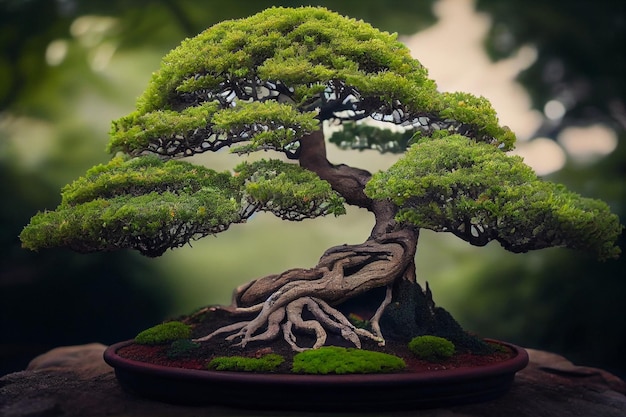The image showcases a beautifully detailed bonsai tree in a well-polished wooden planter, placed upon a flat, brown stone surface. The bonsai has a gracefully curvy trunk with a squiggly set of exposed roots spreading out at its base, surrounded by small green bushes. The tree's numerous tiny branches support bright green leaves, forming a bell-shaped crown. The background, a blur of dappled light filtering through out-of-focus vegetation, gives the impression of a forest setting, though the exact nature—be it a real photograph or a digital creation—remains ambiguous. This artful depiction captures the essence of traditional Japanese bonsai, emphasizing intricate care and meticulous craftsmanship.